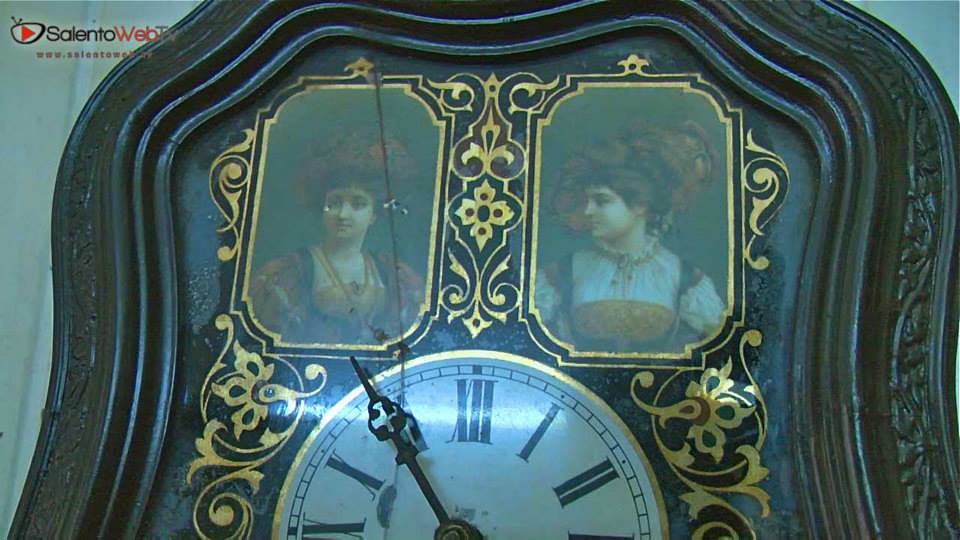This rectangular, horizontally-oriented image appears to be part of an advertisement. The upper left corner features the text "Salento Web" in black and red against a gray background. Dominating the majority of the photo is the ornate top portion of an antique clock. The lower section of the image includes half of the clock's white face bordered in gold, adorned with Roman numerals, and showing a single hand pointing to the 11. Above this clock face lies a black clockplate embellished with intricate gold details. Situated within this decorated frame are two vintage images of women dressed in elegant Victorian attire. Both women, visible from the chest up, wear opulent hats and fancy dresses, further enhancing the antique and nostalgic charm of the piece.